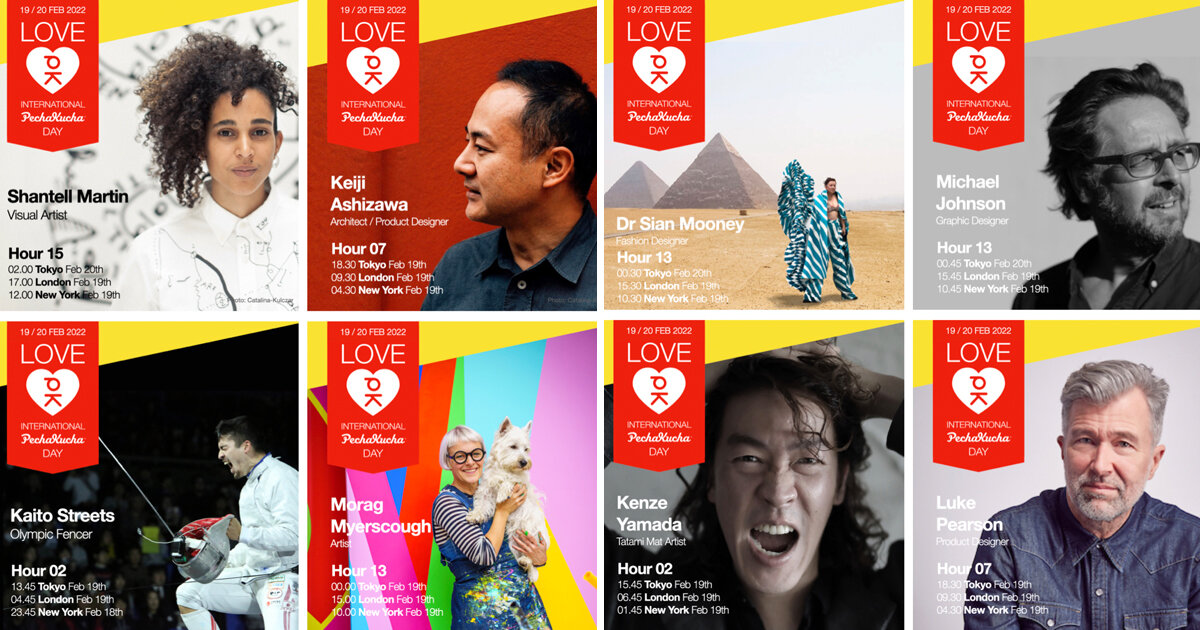This image is a detailed screenshot from a website showcasing eight portraits of individuals arranged in two rows of four. Each portrait is topped with a yellow triangle and a red banner. The banner features white text announcing "Love PK International PechaKucha Day" scheduled for February 19th and 20th, 2022.

- **Top Row (from left to right):**
  1. **Chantelle Martin:** A young woman with curly hair, dressed in white, identified as a visual artist. This portrait is associated with hour 15.
  2. **Keiji Ashizawa:** A man of Asian descent with black hair, attired in a denim or blue shirt, recognized as an architect/product designer. This portrait is marked with hour 7.
  3. **Dr. Sian Mooney:** Seen from a distance, this individual stands before the Great Pyramid on sand, clad in an elaborate turquoise and white striped outfit. This fashion designer’s segment is at hour 13.
  4. **Michael Johnson:** A black and white photograph depicts a man with dark hair, glasses, and a beard, dressed in a black shirt. He is identified as a graphic designer, featured at hour 13.

- **Bottom Row (from left to right):**
  1. **Kaito Street:** A man in a white fencing outfit, holding a helmet and sword. An Olympic fencer scheduled for hour 2.
  2. **Morag Myerscough:** A woman in a blue dress holding a white dog, wearing black-rimmed glasses. Listed as an artist, appearing at hour 13.
  3. **Kenzie Yamada:** A man of apparent Asian descent with black hair, his mouth open as if screaming, wearing a black shirt. Identified as a Tatami mat artist, scheduled at hour 2.
  4. **Luke Pearson:** A man with gray hair and a beard, pale skin, blue eyes, dressed in a button-up denim shirt. Recognized as a product designer, featured at hour 7.

The vibrant and diverse assortment of individuals highlights various professions and global participation for Love PK International PechaKucha Day 2022.